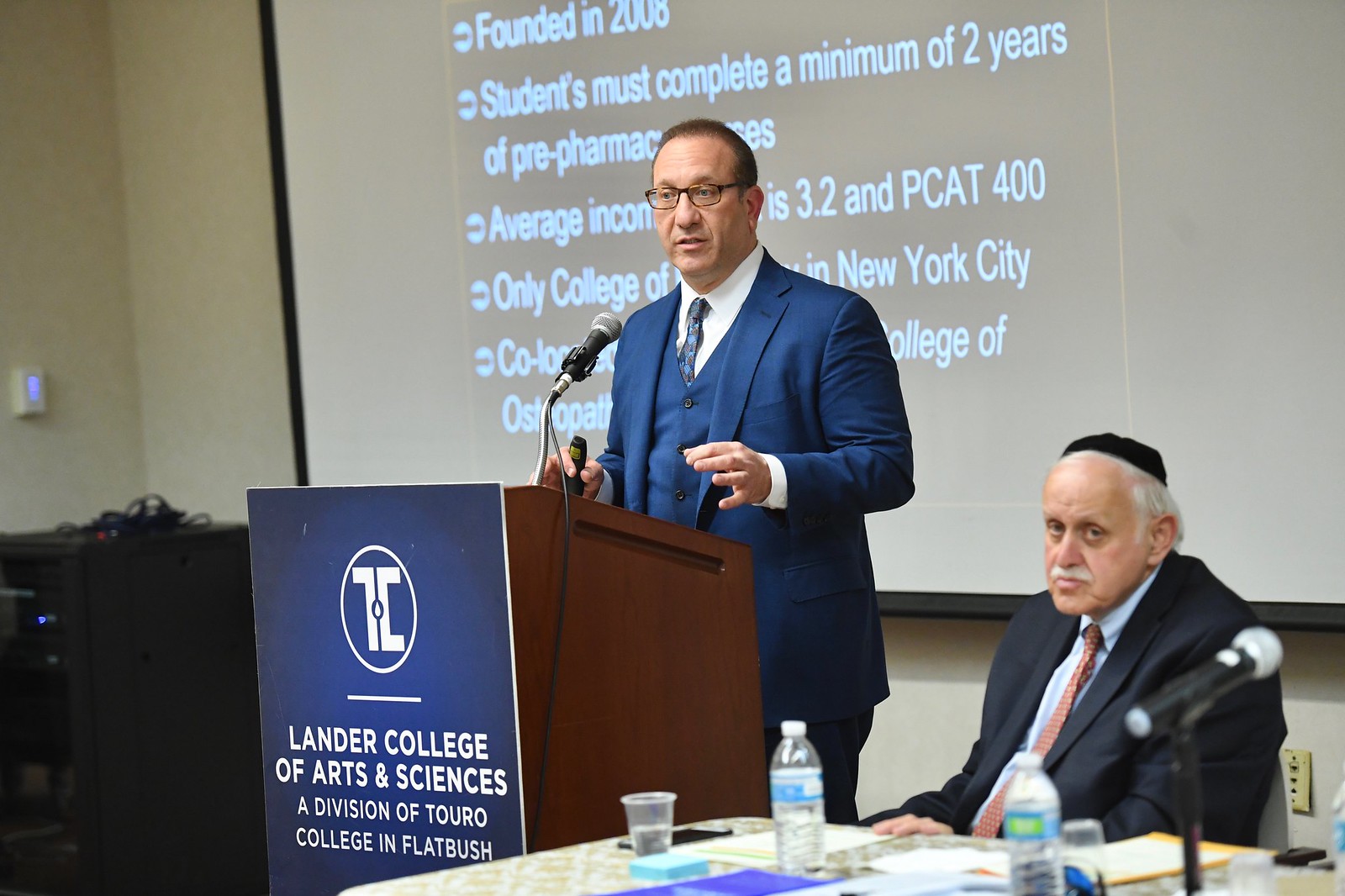In this indoor photograph taken in a professional setting, we see two men who appear to be part of a formal presentation or speech. The primary focus is on the man standing at a wooden podium adorned with a blue sign that reads in white text, "Lander College of Arts and Sciences, a division of Touro College in Flatbush." He is dressed in a sharp blue suit with a white undershirt, a blue vest, and a blue and black tie. This man is speaking into a microphone and is wearing glasses. Behind him, a projector screen displays some details about the college, including "Founded in 2008" and "Students must complete a minimum of two years of pre-pharmacy courses," although his position partially obstructs the rest of the text.

To the right of the podium sits an older man at a table, wearing a black suit jacket, a blue undershirt, and a red tie with yellow spots, along with a black yarmulke on his head. He has white hair and is seated at a white table that holds water bottles, papers, a half-filled cup of water, what seems to be a calculator, and a microphone on a stand. The room itself appears to be a conference or classroom setting, with a white-painted wall and a black desk visible in the background.